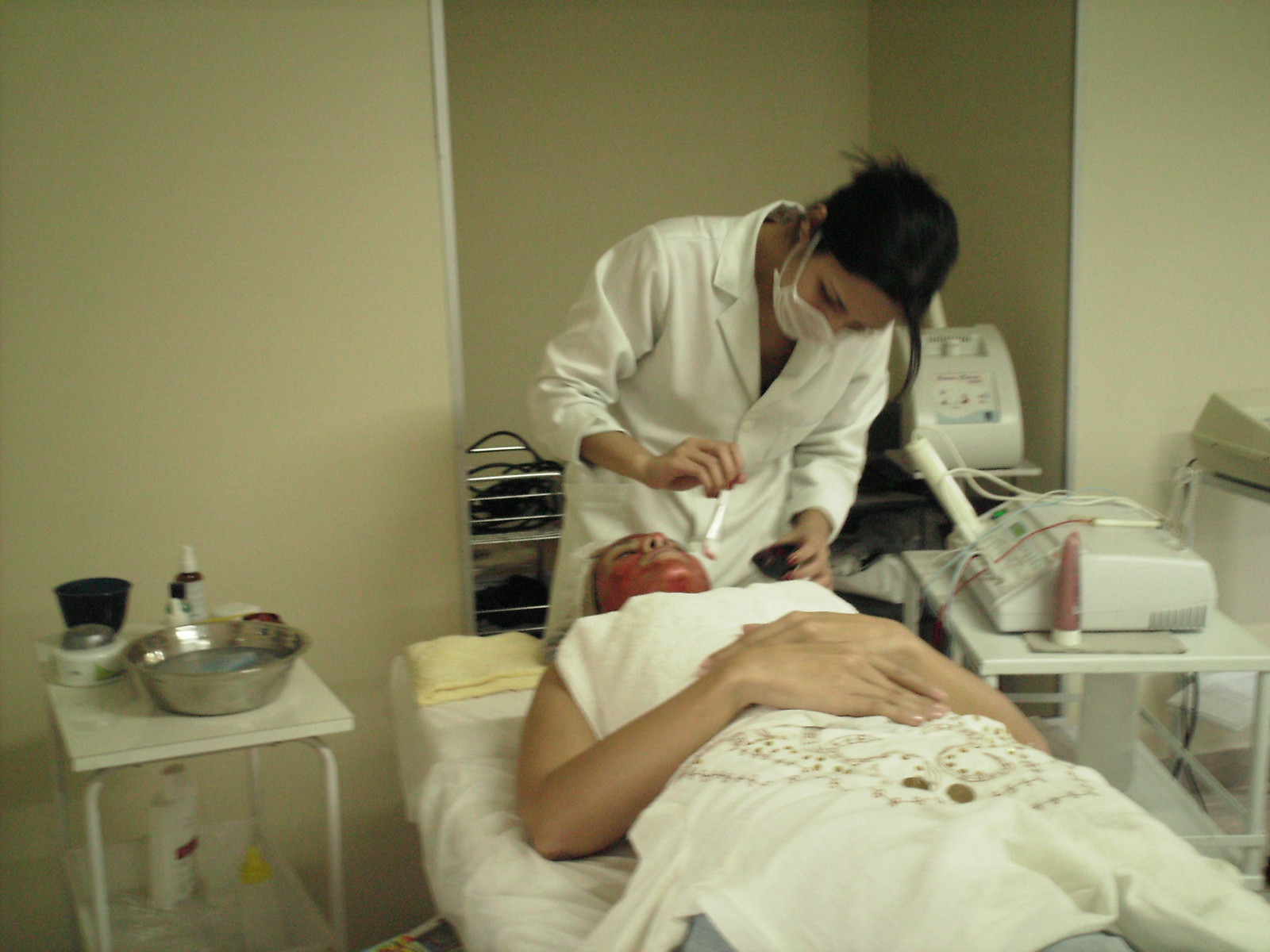In this detailed photograph depicting an esthetician in a treatment room, a client is seen lying on a treatment bed covered with a white sheet, with her hands resting on her abdomen. The client appears to be receiving a facial treatment, evidenced by the esthetician, a brunette wearing a white lab coat and face mask, who is attentively bent over the client. The esthetician is using a white, long-handled brush to apply a red liquid or ointment to the client's face, which appears flushed from the treatment. She holds a small black bowl in her other hand containing the substance she is applying. The treatment room is adorned in beige tones and equipped with various medical instruments. On the right side, there are two apparatuses, including a notable brown tube with a white cap. On the left, a white bedside table hosts a stainless steel bowl, various implements on top, and a bottle underneath. The scene conveys a professional, clinical ambiance dedicated to skincare and treatment procedures.